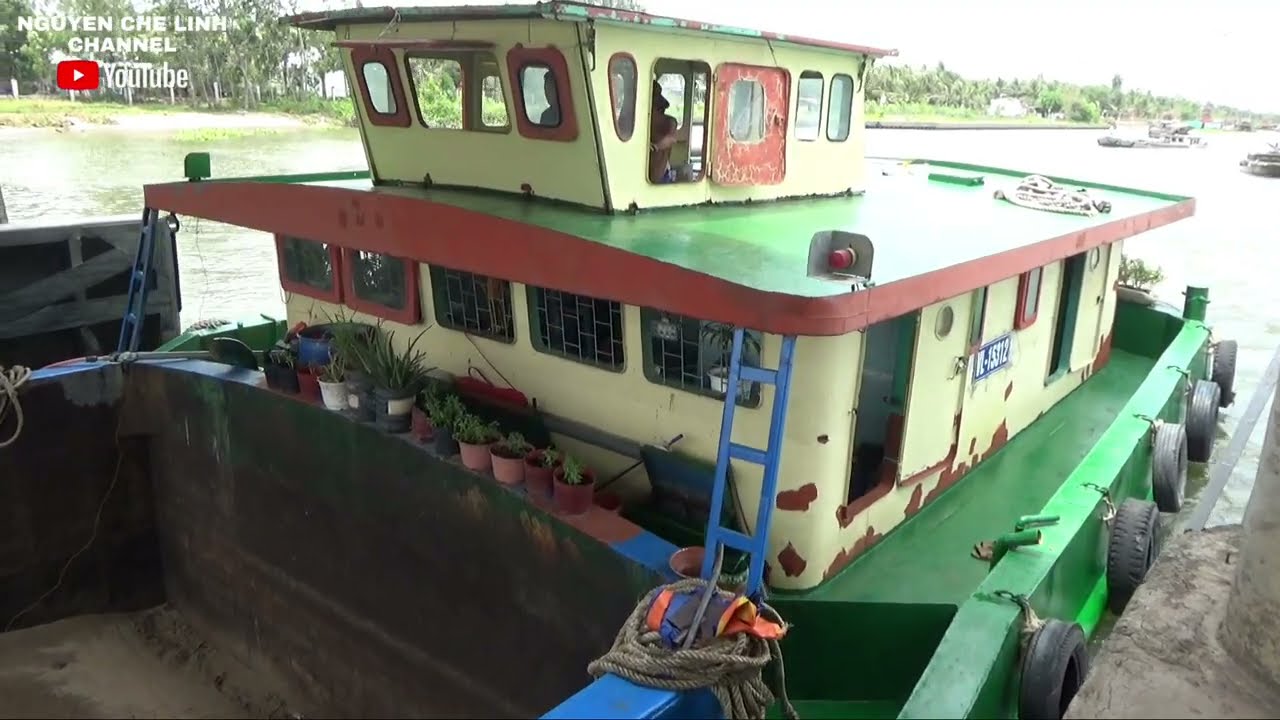In this detailed photograph of a boat moored beside a concrete dock, we see an old, slightly decrepit vessel with multiple levels and distinct features. The camera is angled down the river, capturing the boat illuminated by sunlight, which gives it a pure white appearance due to the camera's exposure settings.

The boat, likely a tugboat, has an exterior marked by green and cream-colored paint, with a deep green floor and lime accents below. The main cabin is a large, square structure with peeling cream paint, revealing burgundy patches beneath. The cabin's roof has burgundy trim and a smaller cream-colored cabin on top, which is likely the pilot's area, complete with windows and a green roof. 

A row of black tires is strategically tied to the side of the boat facing the dock, serving as bumpers to prevent damage when docking. The front of the boat contains a bucket-like area with rusted metal, and just beyond it, there are neatly arranged potted plants with vibrant greenery on display. Additionally, a small blue ladder is seen on the right side, providing access to the upper levels.

In the distance, another similar boat floats on the river, and the opposite bank is lined with lush trees and houses. The photo also features the text "Nugent Chin Lin Channel YouTube" in the upper left-hand corner, suggesting a YouTube channel associated with the image. The overall scene is rich with detail, capturing both the character of the boat and its serene surroundings.